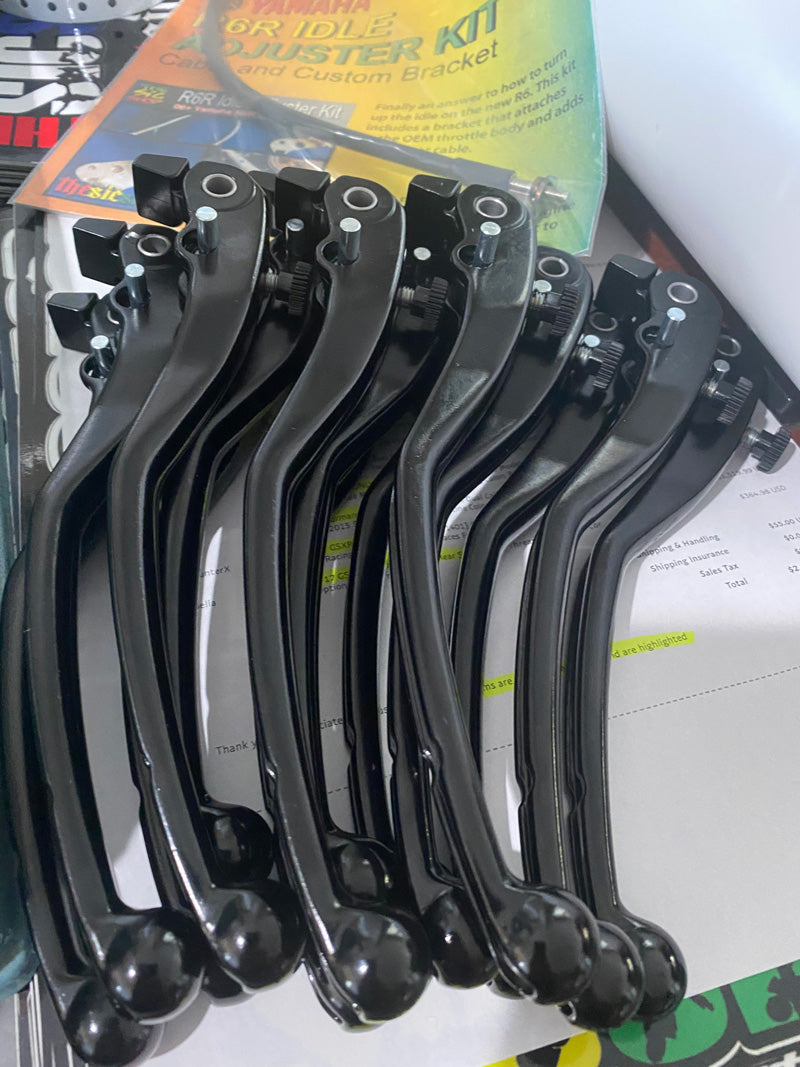This photograph features a collection of about a dozen black metallic tools, prominently displayed as they hang from pegs. Each tool has a distinctive design with a round ball at the bottom, which is attached to a slender metallic neck. This neck extends into a boxy, curved top section with a metallic silver thread or nut inset. Additionally, beneath this threaded area, there is a hole used to mount the tools onto metal dowels. These tools occupy most of the frame, arrayed in a manner that suggests they could be components for exercise equipment or some specialized mechanical use.

Beneath the tools lies a white piece of paper adorned with black printed text such as "shipping and handling," "shipping insurance," "sales tax," and "total," with portions of the text highlighted in yellow. In the background, a brightly colored paper booklet with an orange, yellow, and green gradient cover is visible. This booklet features the title "Yamaha 6R Idle Adjuster Kit Cable and Custom Bracket," along with an indecipherable section of black text and a demonstration image on the bottom left.

The setting appears to be a casual environment, likely inside someone's house, with the tools seemingly organized and awaiting use or installation.